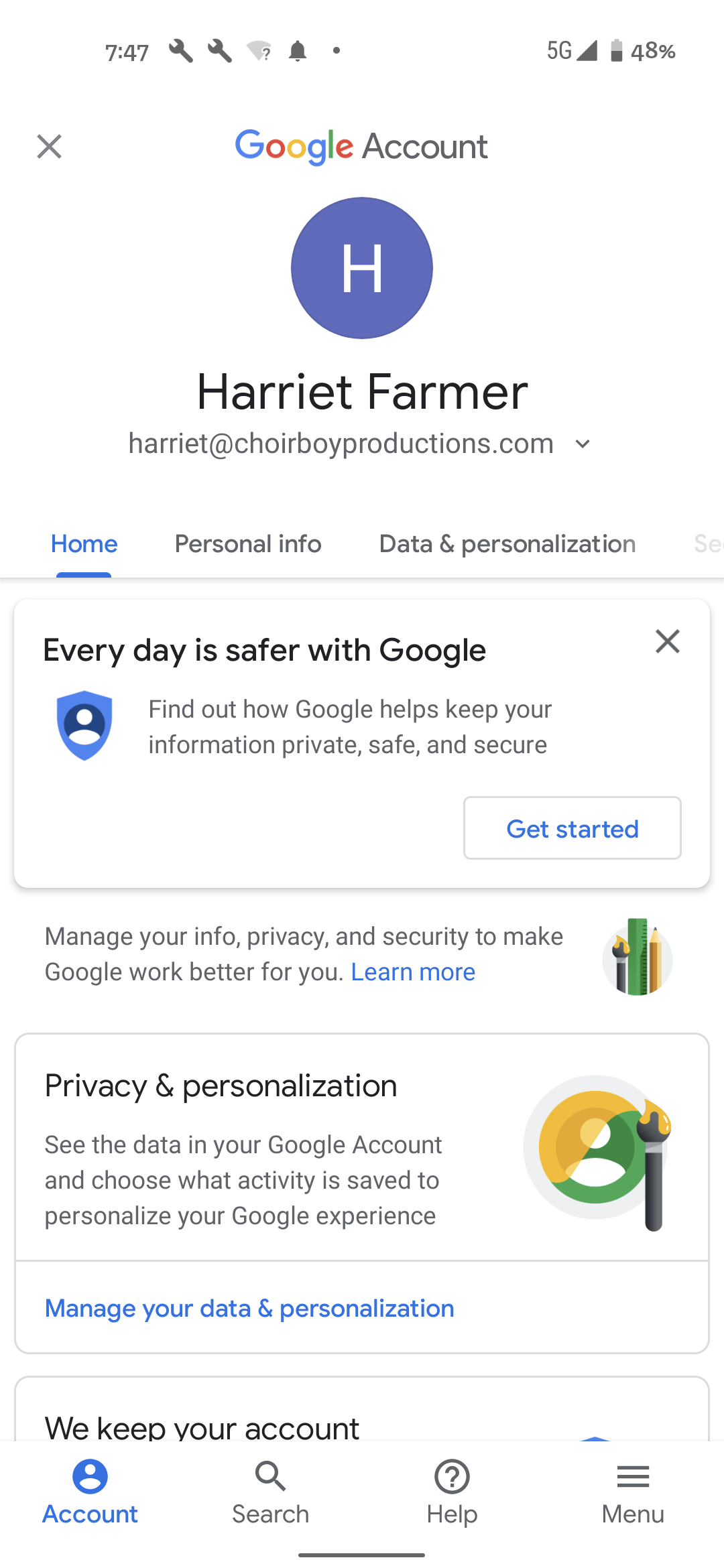A screenshot captures an individual examining their Google account on their smartphone. At the top, the time is displayed as 7:47. The status bar shows two side-by-side wrench icons, a Wi-Fi symbol with a question mark overlay, a bell icon with a dot next to it, a 5G indicator with a full signal bar, and a battery icon indicating 48% charge. To the left, a gray 'X' is visible. 

Beneath this, the title "Google Account" is displayed in gray, followed by the colorful Google logo. Below, there is a lavender circle with a white capital "H" inside, and the name "Harriet Farmer" is prominently shown in large text. Below her name, her email address "harriet@choirboyproductions.com" is displayed.

Underneath, a menu lists "Home," "Personal Info," and "Data and Personalization," with "Home" selected and highlighted in blue. 

A pop-up message states, "Everyday is Safer with Google. Find out how Google helps keep your information private, safe, and secure," and includes a "Get Started" button. A small badge overlays behind the user icon. Below, the message "Manage Your Info, Privacy, and Security to Make Google Work Better for You" is followed by a "Learn More" link and pencil icons on the right.

Further down, a section titled "Privacy and Personalization" features a user icon next to a paintbrush dipped in yellow paint with a yellow stripe across the image. It provides information on how to see the data in your Google account and select activities to personalize your experience, and includes a blue "Manage Your Data and Personalization" button.

At the bottom of the screen, buttons labeled "We Keep Your Account," "Account Search," "Help," and "Menu" are visible.